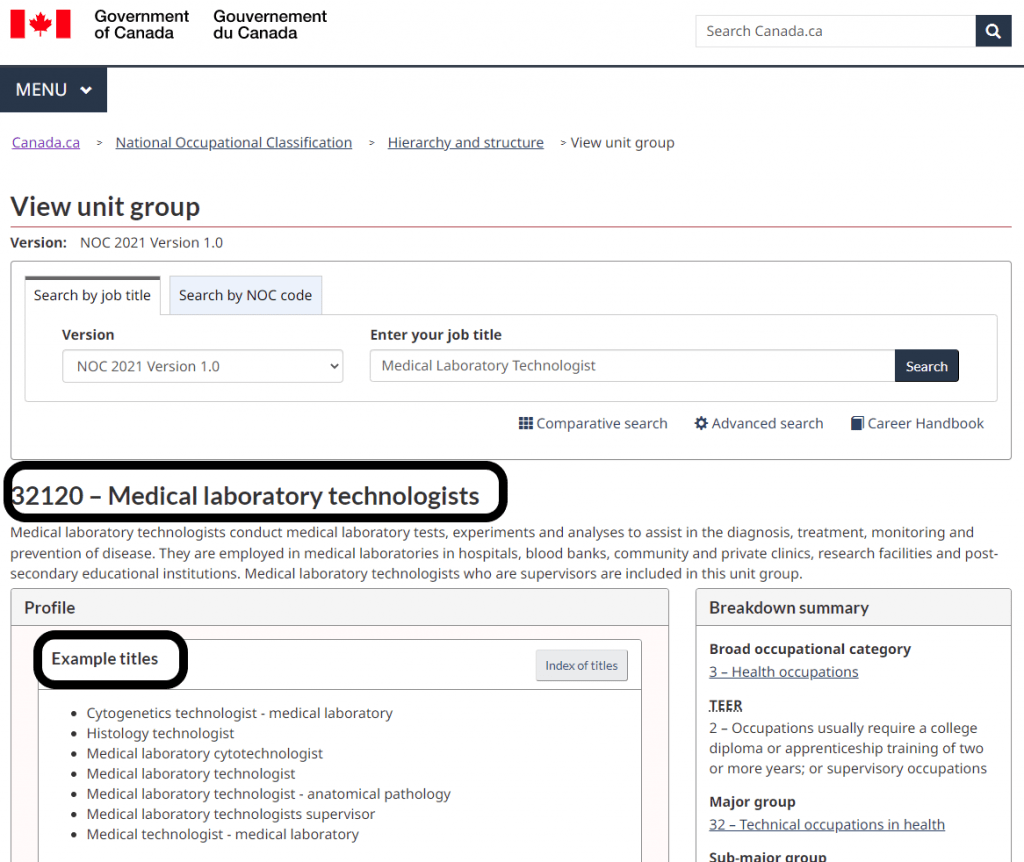The image is a vertical screenshot from a Canadian government website, likely accessible on smart devices and computers. The upper left corner prominently features the red maple leaf Canadian flag, accompanied by the text "Government of Canada" in black. Adjacent to this is the French translation, "Gouvernement du Canada." On the upper right, there's a search bar labeled "Search Canada.ca," complete with a magnifying glass icon.

On the upper left, beneath the flag, there's a menu button. The interface highlights various clickable options, including "Canada.ca," "National Occupational Classification," "Hierarchy and Structure," and "View Unit Group," with the latter option bolded for emphasis. Below this menu, the page lists version information and features a dropdown menu for selecting different versions.

Users can enter their job title or NOC (National Occupational Classification) code into a search field, which in this case, is pre-filled with "Medical Laboratory Technologist." A search button is available for initiating the query. Additional search options include "Comparative Search," "Advanced Search," and "Career Handbook."

On the lower left side of the image, "32120 Medical Laboratory Technologist" appears within a dark black rounded box. Beneath this, there is a descriptive blurb about the profession. The page also includes sections for "Profile Example Titles," featuring indexed titles in another boxed layout. The screenshot further elaborates on the classification hierarchy with a breakdown summary encompassing the broad occupational category, tier, major group, and sub-major group.